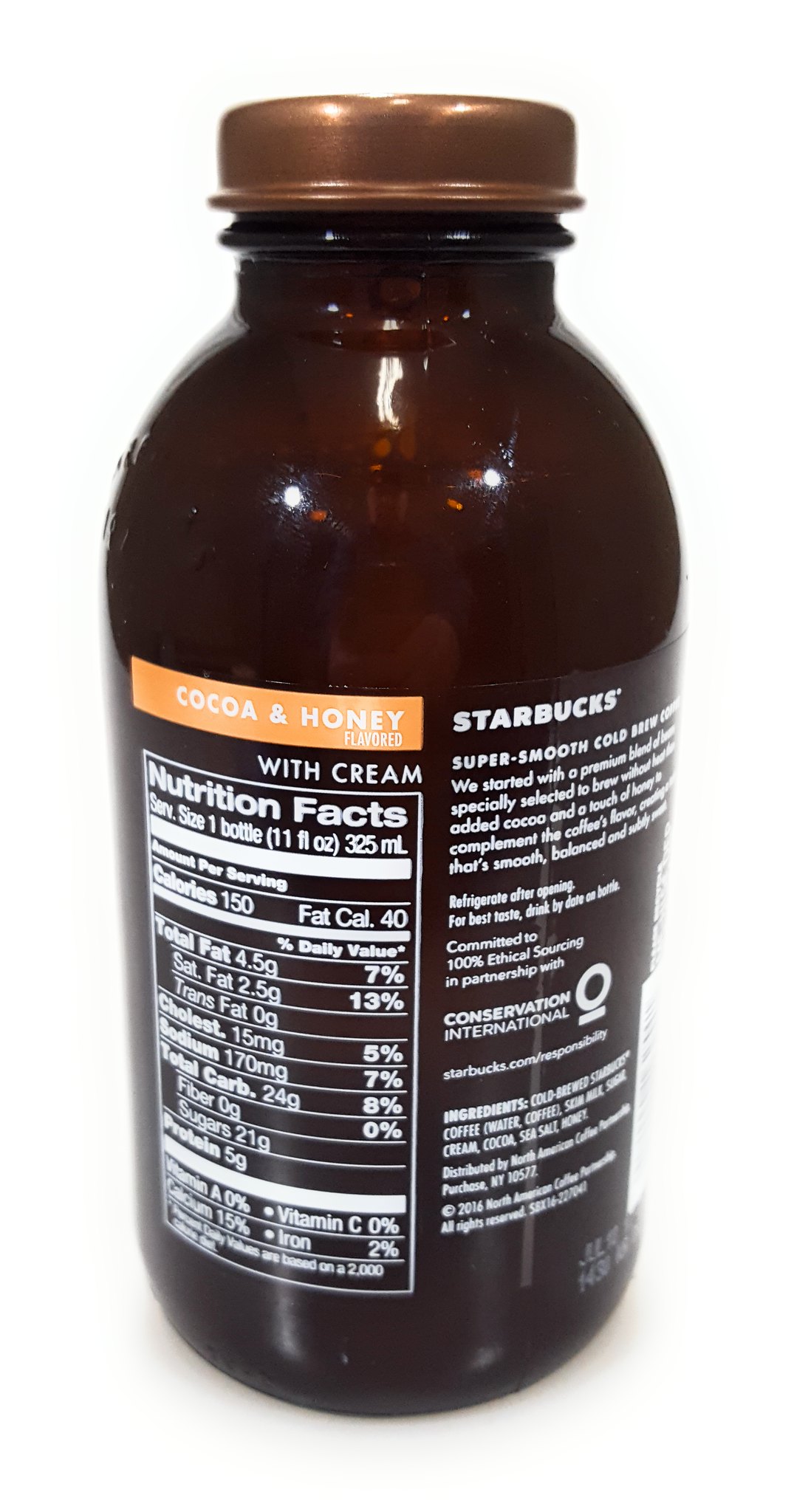This image features a glass bottle against a completely white background. The bottle is brown and prominently displays a label. On the right-hand side of the label, the word "Starbucks" is visible. The label also includes a partially obscured text that reads "super smooth" followed by unreadable text. Additionally, the label states "Cocoa and Honey with Cream" in white letters placed inside an orange banner. The bottle provides nutrition facts, indicating it contains 150 calories, with 40 of those calories coming from fat. It also notes that it is an 11-ounce bottle and that the saturated fat content is 13%.